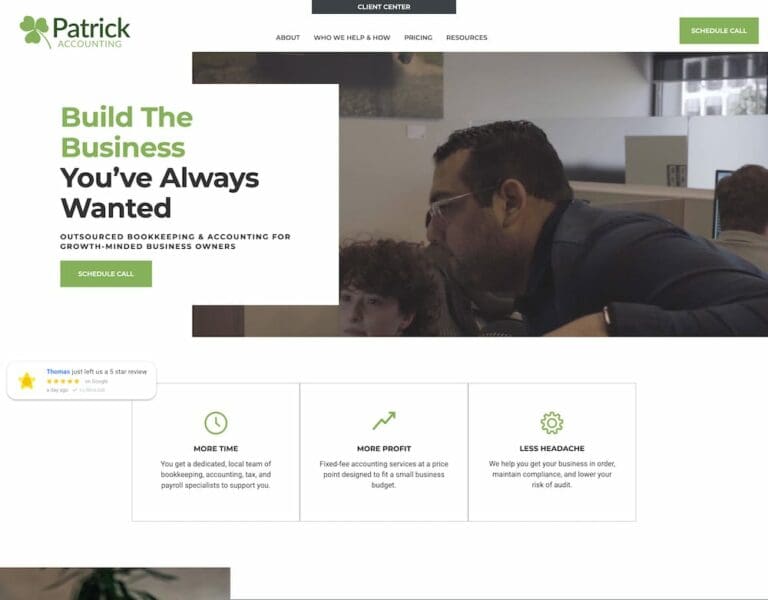This screenshot from the Patrick Accounting website captures its visually appealing and informative design. The company's logo, a three-leaf clover, is prominently displayed in the top left corner. Adjacent to the logo, the navigation bar extends across the page, featuring tabs labeled "About," "Who We Help," "How," "Pricing," and "Resources." Above this, a sleek black stripe contains the "Client Center" link. On the far right of the navigation bar is a vibrant green "Schedule Call" button. 

Dominating the main content area below the header is a large image of a man and woman looking intently at a computer screen, suggesting a collaborative and productive atmosphere. To the left of this image is a small white box with bold text, presenting the motivational headline: "Build the Business You've Always Wanted." Complementing this header is another green "Schedule Call" button directly below.

Further down, the page is divided into three sections, each highlighting a distinct benefit of the service. The first section, titled "More Time," features a green clock icon and a brief description below. The middle section, "More Profit," displays an icon of an ascending line graph, while the third section, "Less Headache," is marked by a gear icon. Each section provides a concise explanation to support the respective titles.

To complete the design, a small rating bubble from a client named Thomas is displayed in the top left corner, boasting a perfect rating of five yellow stars. The entire page is set against a clean, white background, ensuring that the content remains clear and legible.